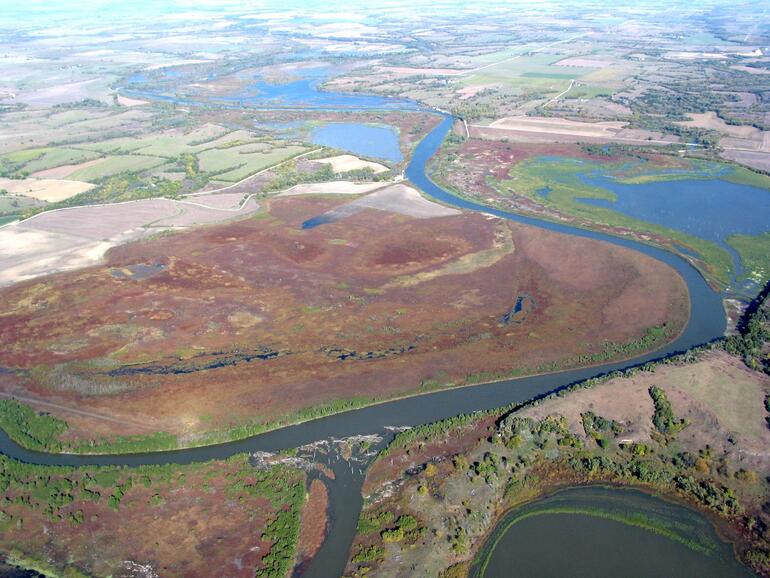The image showcases an aerial view, likely captured from a plane or drone, depicting an expansive stretch of flat land characterized by natural waterways meandering through the landscape. The terrain appears to be a mix of farmland and wetlands, hinting at recent flooding with visible large puddles and water spillovers beyond the river's usual path. This intricate network of rivers and possibly small lakes intricately intertwines with the land, creating a patchwork of diverse colors and textures. The fields are a blend of beige, light red, and green, suggesting varying types of vegetation and land use. In the distance, approximately a mile or two away, hints of trees and roads can be discerned, their details softened by the altitude. The water's hue shifts from a bluish tint, likely reflecting sunlight, to a grayish tone in the foreground, indicating possible sediment or murkiness. Scattered around the edges and within the landscape are clusters of trees, enhancing the scene's natural beauty and complexity.